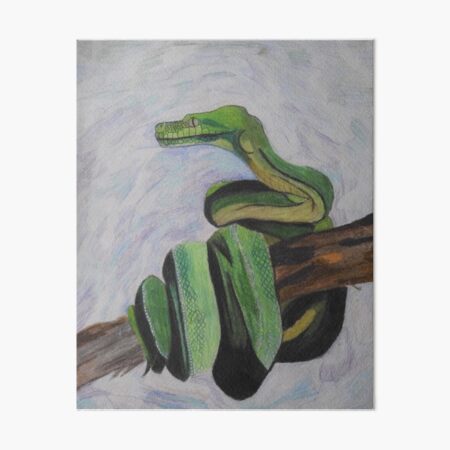The image is an intricately drawn illustration, possibly created with colored pencils, depicting a small green snake coiled multiple times around a thick, dark brown wooden branch located in the lower part of the picture. The background features swirling patterns in shades of white, blues, purples, and grays, creating a cloudy, almost ethereal atmosphere. The snake's upper body and head rise above the branch, facing left. Its green scales are vivid and detailed, transitioning to a yellow tone on the belly and throat. The eyes are strikingly yellow with vertical black slits, adding to its realistic appearance. Shadows are subtly rendered, particularly under the snake's body where it wraps around the branch, adding depth to the scene.